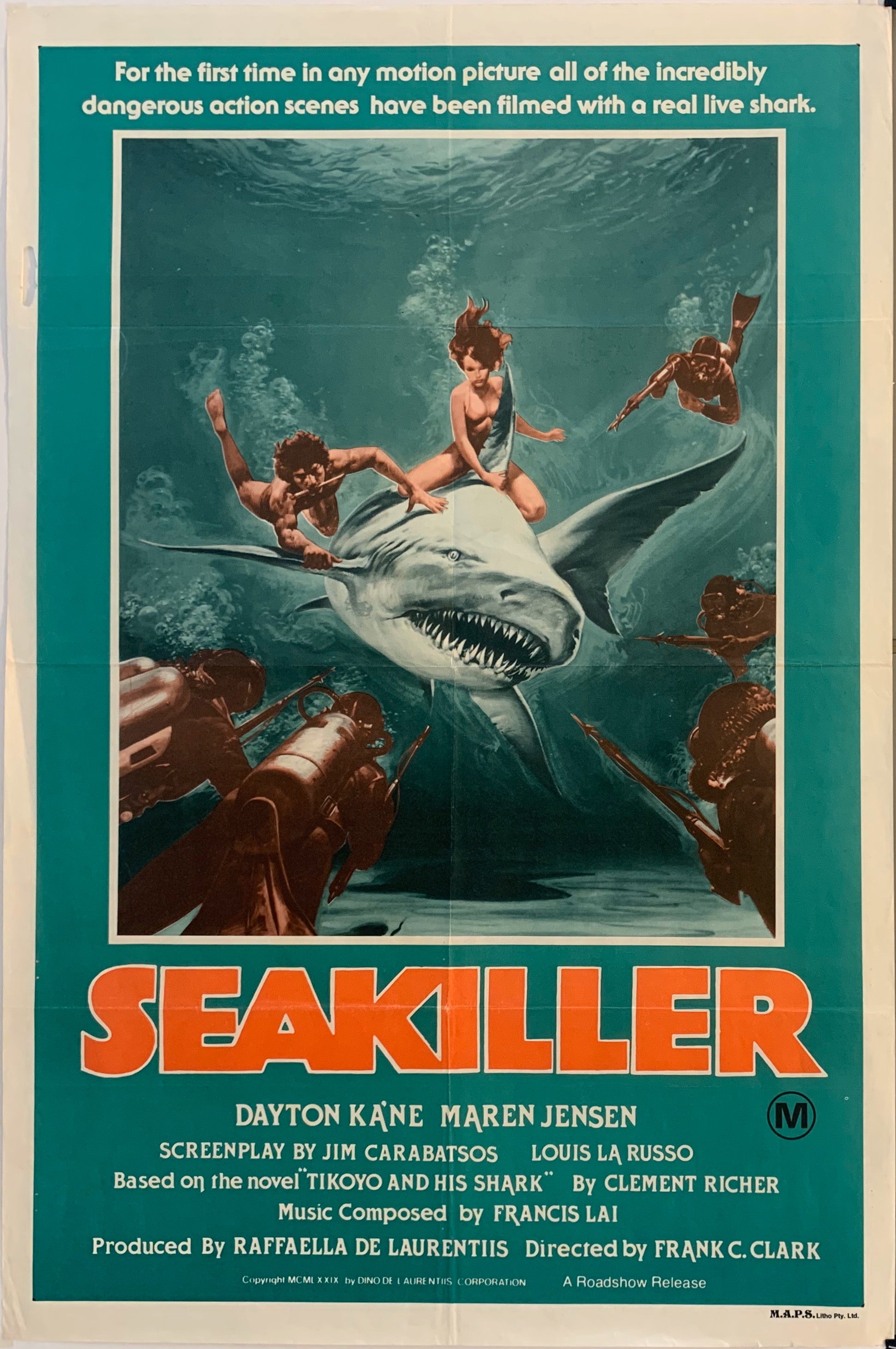This detailed movie poster features an illustrated drawing occupying the top two-thirds of the image. Dominating the center is a large gray shark with its mouth open, revealing long, menacing teeth. Clinging to the shark, a man with brown hair has a knife in his mouth and is gripping one of the shark's fins while partially riding its back. On top of the shark, a woman with brown hair straddles its dorsal fin. Both figures appear almost naked and are underwater, surrounded by approximately seven divers in black suits equipped with oxygen tanks and harpoons, all rendered with a brownish tint as if viewed through an old filter.

The bottom third of the poster features the title "Sea Killer" in bright orange, bold letters, followed by smaller white text providing movie information, such as actor credits and production details. The backdrop of the poster is a dark teal color, which contrasts with the vivid illustration. Crowning the top border, a white inscription proclaims, "For the first time in any motion picture, all of the incredibly dangerous action scenes have been filmed with a real-life shark," emphasizing the use of live-action sequences involving the shark. This vintage-style design evokes a sense of nostalgia, suggesting the film's production era might hail from several decades past, potentially the 1950s or 1960s.